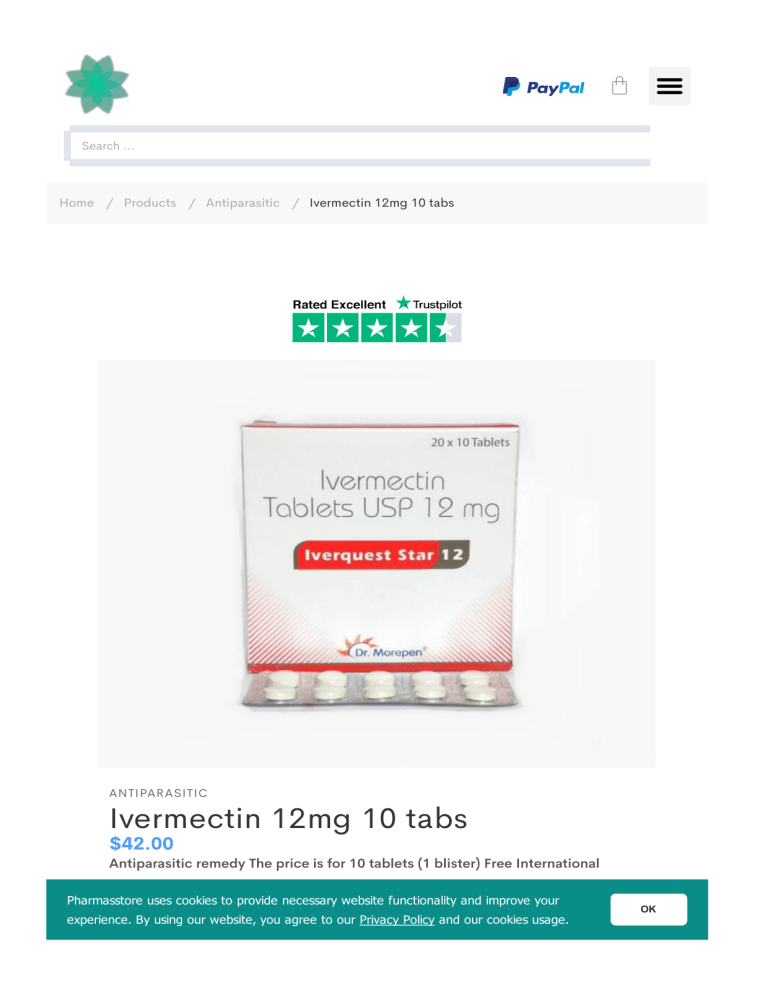The screenshot captures a webpage from an online store called "Spasma Store." In the top right corner, the PayPal logo is prominently displayed alongside icons resembling a padlock and an options menu. Directly below, there is a search bar for site navigation.

The main header of the page reads: "Home > Products > Anti-Parasitic," indicating the item's category. The highlighted product currently being viewed is "Ivermectin, 12 milligram, 10 tablets." 

Underneath the header, a 5-star rating system shows the product's rating as 4.5 out of 5 stars, reflecting high customer satisfaction. The product image displays a white box with red trim at both the top and bottom edges. The text on the box states "Ivermectin Tablets USP, 12 milligrams." In the top right corner of the box, it reads "20 x 10 Tablets," and under that, the product name is identified as "Iverquest Star 12." Finally, at the very bottom, "Dr. Morphine" is noted, likely the manufacturer or endorsing entity.

The product is listed for sale at $42, described as an "Anti-Parasitic Remedy." The price covers 10 tablets, and the offer includes free international shipping for one blister pack. 

At the bottom of the page, the footer includes a message about cookies: "Spasma Store uses cookies to provide necessary website functionality," prompting users to accept cookies for enhanced browsing experience.